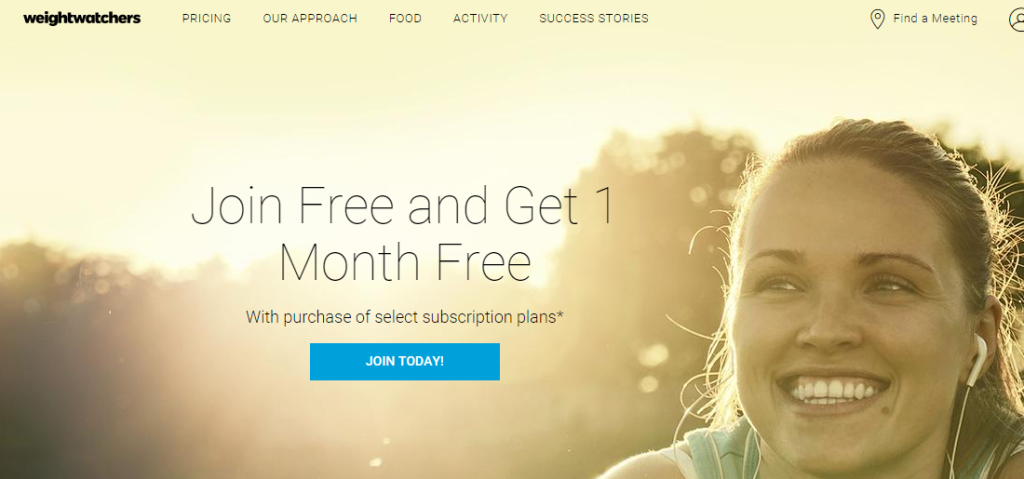The image showcases a banner from a Weight Watchers website. At the top, "weight watchers" is written in bold, black lowercase letters. Adjacent to it is a horizontal menu in lighter print and all capital letters, listing: PRICING, OUR APPROACH, FOOD, ACTIVITY, and SUCCESS STORIES. Continuing to the right, there's a location icon followed by the words "Find a meeting" with uppercase initial letters.

Below this header, the main image features a sepia-toned outdoor scene with a sky and trees in the background. On the right side of the image, there's a girl with her hair pulled back, shown from the chin upwards, with part of her right shoulder visible. She’s wearing earbud-style headphones. Next to her, in larger, thinner text, it reads: "Join free and get one month free with purchase of select subscription plans," followed by an asterisk. At the bottom of the image, a blue banner contains the text "JOIN TODAY!" in all capitalized, white print.